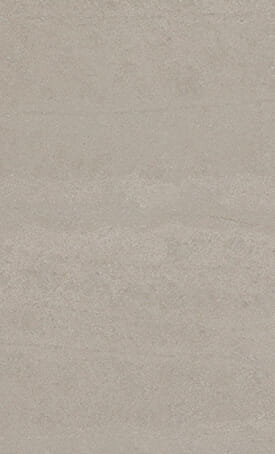This image is a simple, rectangular background with a light gray color and subtle textural details that make it somewhat reminiscent of smooth concrete or a wooden pattern. The background has a wave-like texture with faint lines running through it, providing an ink-like quality to the appearance. The image is taller than it is wide and contains no prominent features such as people, text, or drawings, making it resemble a plain, painted piece of paper or wall. With its minimalistic design and subtle textures, this image could easily be used as a wallpaper.